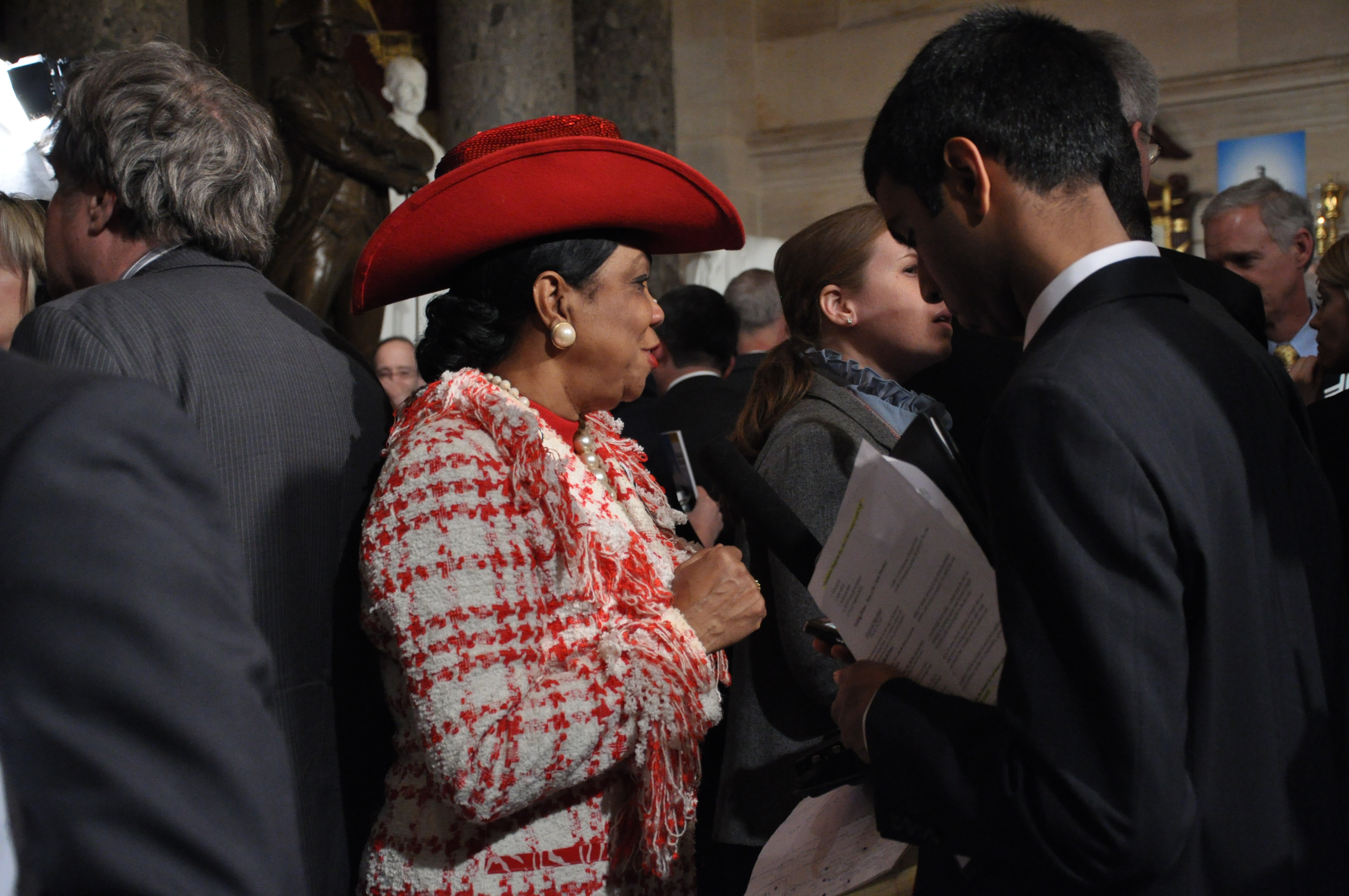This is a detailed color photograph taken indoors, capturing a large gathering of men and women, all of whom appear to be over 40 years of age. The scene is quite dense, with people standing very close to each other, almost touching, creating a slightly claustrophobic atmosphere due to the crowded space. 

The central focus of the image is an African American woman positioned just left of the center. She stands out vividly in her bright, eye-catching attire. She wears a large red cowboy-style hat, prominent pearl earrings, and a red and white jacket adorned with fringe, paired with a red shirt underneath. Her long hair is meticulously braided, rolled, and pinned to the back of her neck in an elegant style. Her right arm is bent with her hand slightly in front of her body as she faces to the right, engaging in a conversation with a younger man holding some papers.

Flanking her, partly visible from behind, are two men in suits. One to her left, with short grayish hair, is facing slightly away from her. To her right, another man with short black hair, is similarly turned away, revealing his back and the side of his suit. In between her and this man, and slightly further into the background, there's another woman, who is also facing to the right but less prominently visible.

The room is bustling with people, most of whom are engaged in conversation and are dressed in business attire. The setting, filled with various background elements like walls and possible statues, suggests it might be a government building. The woman in red, possibly a representative, gives the impression of being in a position of authority or significance, perhaps even in the midst of an interview or discussion.